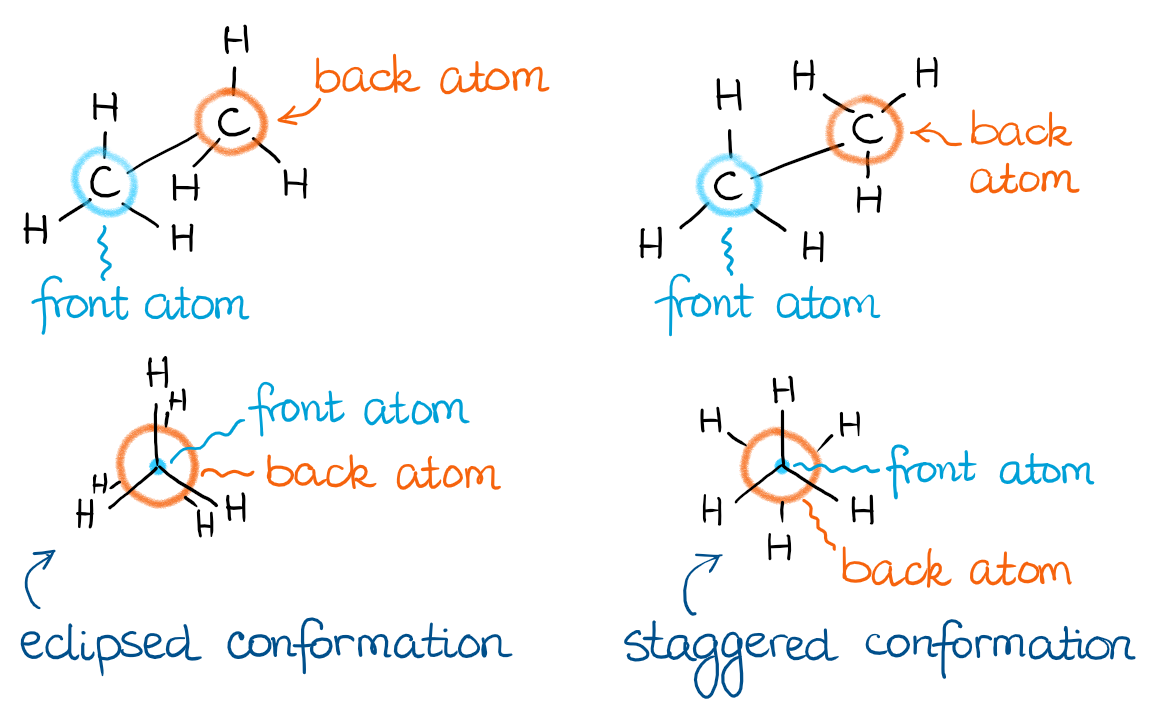This detailed scientific diagram, likely designed for educational use in a classroom or laboratory, illustrates the concepts of eclipsed and staggered conformations of molecular structures. The left side of the diagram features the eclipsed conformation, labeled at the bottom in blue lowercase letters. Here, hydrogen atoms (H's) are positioned at the top, left bottom, and right bottom sides of the structure. A blue squiggly line points to text reading "front atom," and a red squiggly line points to text reading "back atom." Additionally, arrows and C labels emphasize the front and back carbon atoms within the hydrogen configuration. The right side mirrors this layout but illustrates the staggered conformation. Similar hydrogen atom arrangements are shown surrounding what resembles a clock diagram, with annotations labeled "front atom" and "back atom." The diagram prominently uses colors such as blue and orange to highlight key components and connections, enhancing the visual distinction between the front and back atoms (circled in respective colors) and their spatial arrangements. Despite its complexity, this diagram serves as a crucial visual aid in understanding molecular conformations in chemistry.